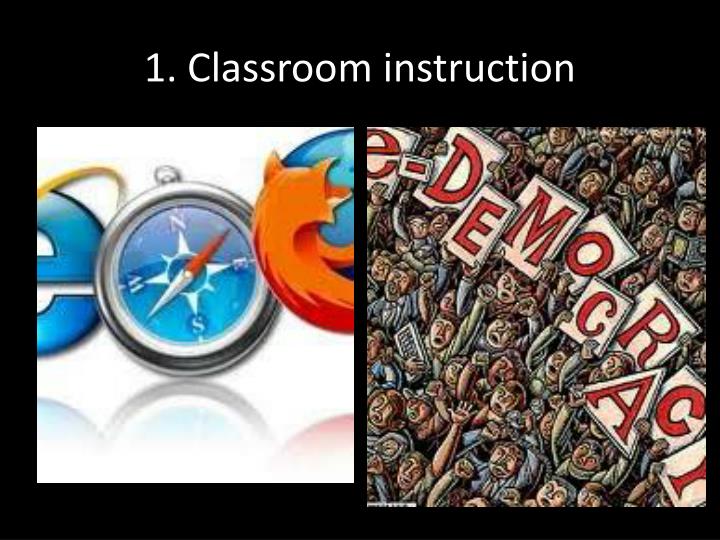The slide features a black background with white text at the top, reading "1 period CLASSROOM INSTRUCTION." Below the text are two distinct images. The left image displays three logos for web browsers—Internet Explorer, Safari, and Firefox—arranged from left to right on a white background, with their reflections visible below them. The Internet Explorer logo is a blue "E," Safari is represented by a compass with a blue background and silver circle, and Firefox features an orange fox encircling a blue globe. The right image depicts a cartoonish crowd of people, all animatedly holding up white signs with red lettering that spells out "E-DEMOCRACY," with some people shouting and raising their fists in the air.